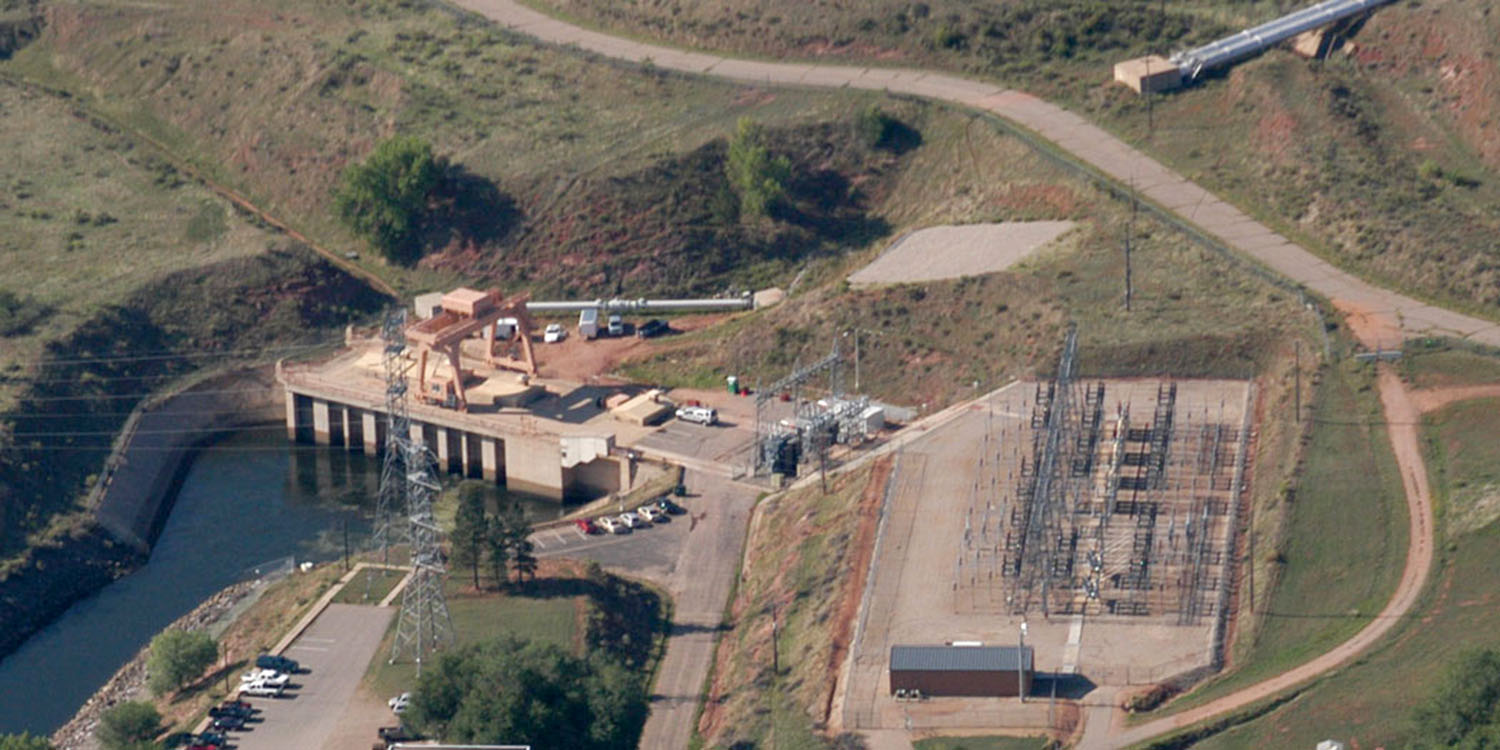This aerial photograph captures a sprawling landscape featuring a power station situated on a sloping hill. At the center of the image, you can see tan cement structures and various power units placed on level terrain. Adjacent to the power station, there's an organized parking area with a few cars parked, indicating some level of activity. Toward the left side of the image, a dark blue water body is contained by a constructed wall, offering a tranquil contrast to the industrial elements. Two large cell towers stand on flat ground near the parking area. Scattered throughout the scene are dirt roads, patches of grass, several trees, and a long metal pipe. The surrounding area appears rural and sparse, lacking urban features like stores or dense infrastructure, emphasizing the isolated setting of this facility.